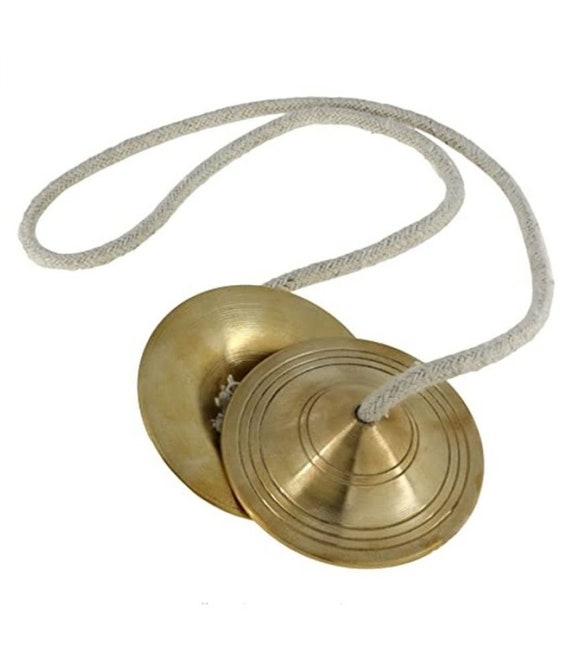This image features a pair of brass castanets connected by a light gray, woven rope with a slightly fuzzy texture. The castanets, which overlap, appear dulled with a muted gold hue, and the one on top showcases intricate, concentric engravings in five circular lines. The top castanet has a domed shape, leading to a hole where the rope passes through. The bottom castanet, partially visible and upside down, lacks any embossing. The rope, approximately a quarter-inch thick, securely tethers the two instruments together. The photograph is isolated against a white backdrop, emphasizing the detailed craftsmanship and structure of the brass castanets.